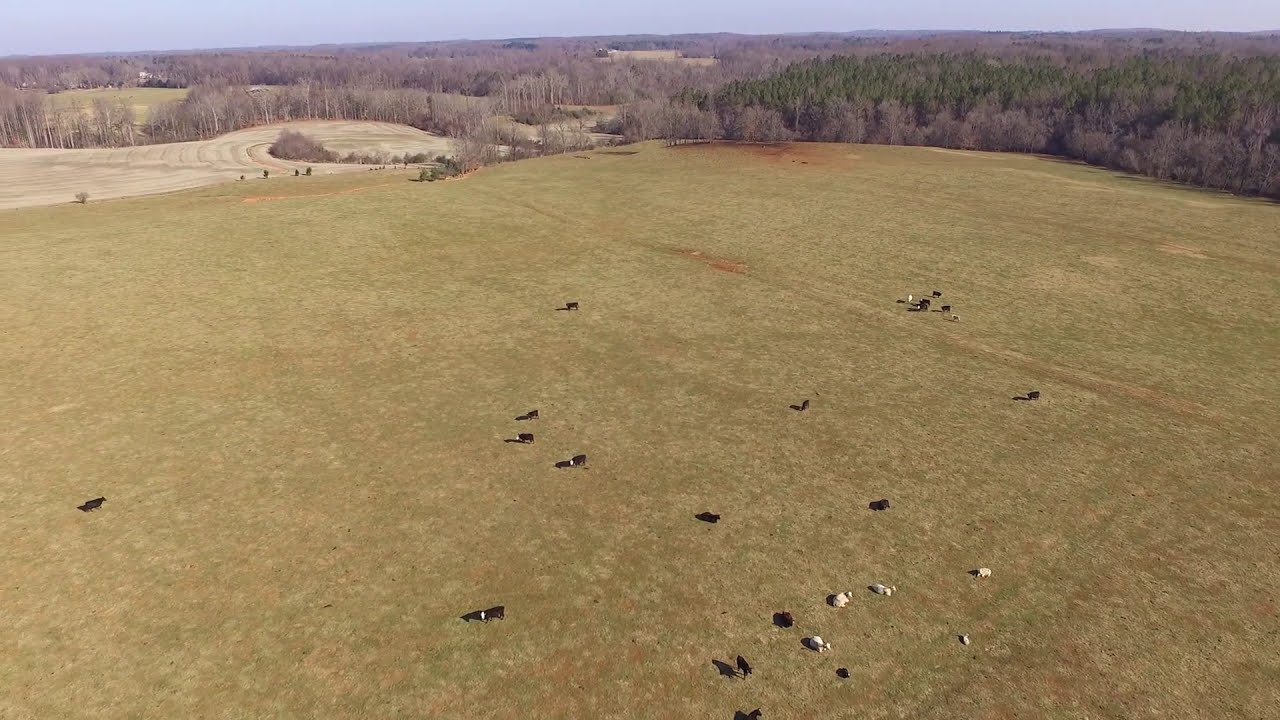The aerial image showcases a sprawling countryside field with a mosaic of light green and brown hues. This pastoral scene features numerous cows, both brown and white, scattered predominantly across the bottom center of the image, casting elongated shadows under the sun. Towards the top, the land appears more barren, with vast stretches of grassland and patches of dark soil and cut grass forming distinct patterns. In the distance, a tree line borders the field, with seemingly dead trees interspersed with clusters of green foliage. The top right corner reveals a dense green woodland, contrasting with the largely bare trees, which indicate a winter setting. On the top left, some distant buildings are faintly visible against the flat landscape, all beneath a clear blue sky stretching across the upper part of the photograph.